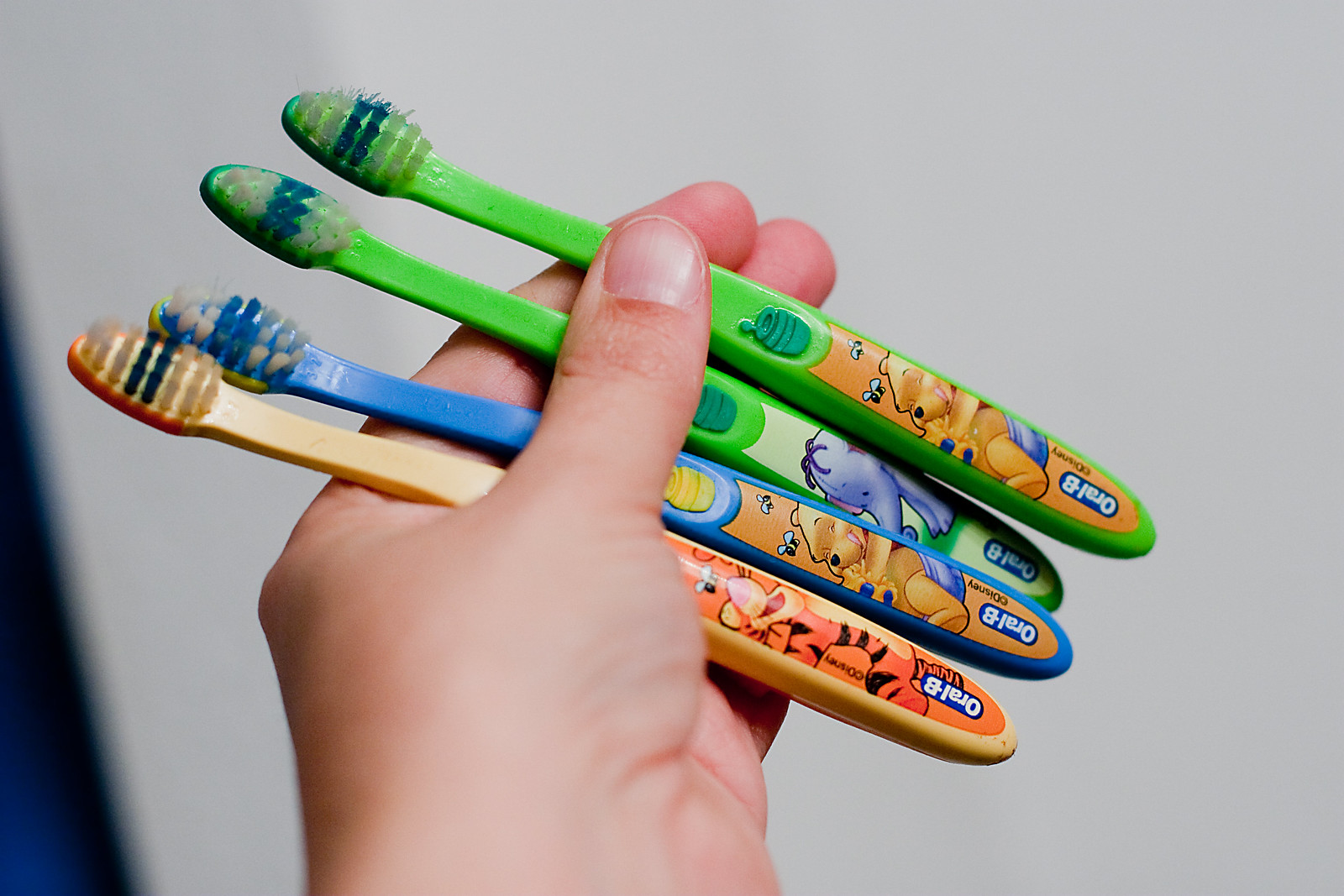In this photo, set against a gray wall background, an adult's well-maintained hand with fair skin is outstretched, holding four children's toothbrushes. These toothbrushes are designed with beloved cartoon characters from Winnie the Pooh and are all made by Oral-B. The first toothbrush is yellow-orange, featuring Tigger, with tan and black bristles. The second is blue, adorned with Winnie the Pooh and has blue and white bristles. The third toothbrush is green, showcasing Eeyore with blue and white bristles. The fourth one is also green, featuring Winnie the Pooh, and has white and blue bristles. Each toothbrush handle has raised decorations resembling a honeypot. Despite their color and character variations, all toothbrushes appear slightly used, instilling a sense of nostalgic familiarity.